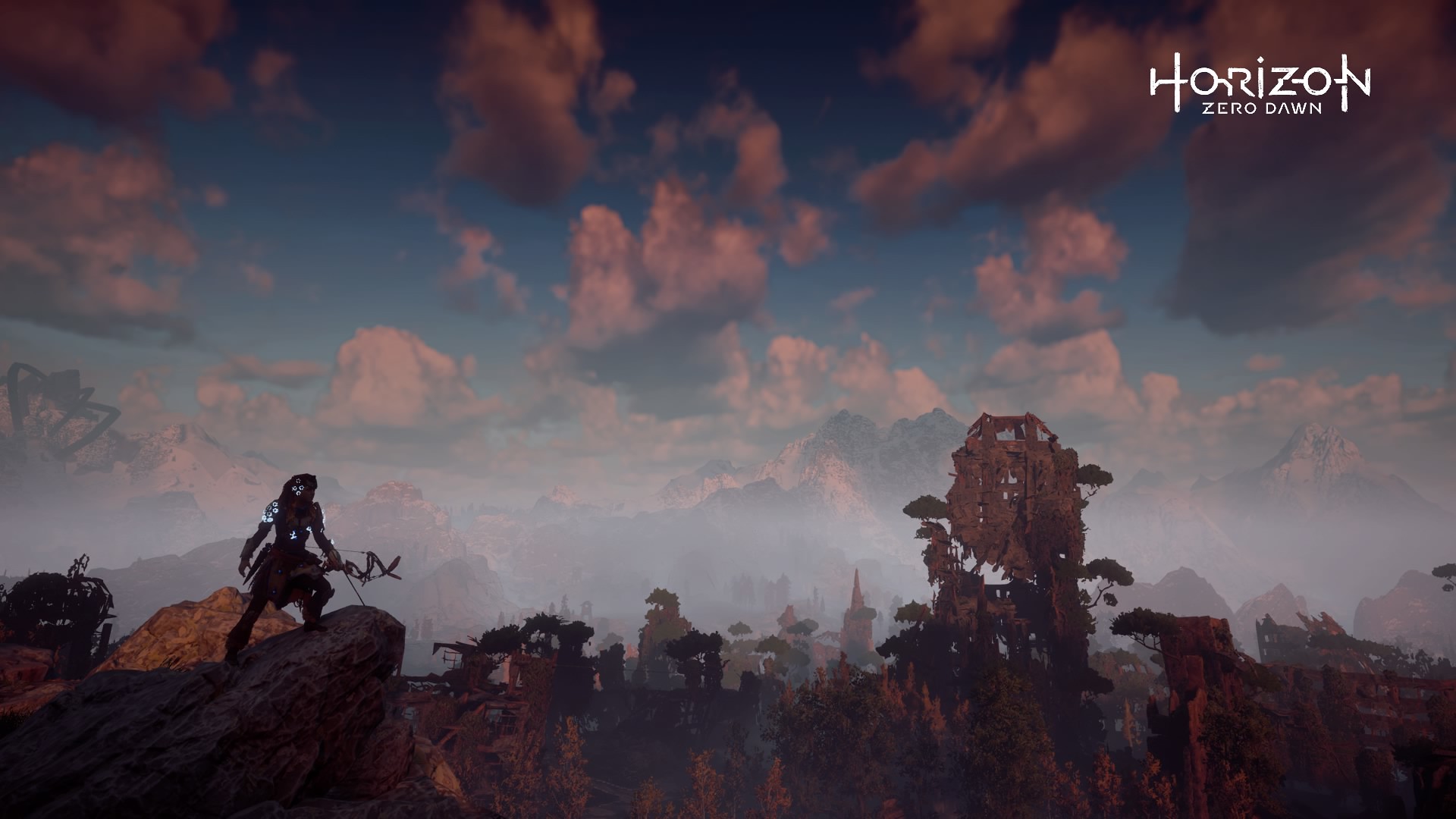This is an intricate digital image of the video game "Horizon Zero Dawn." At the top center of the image, the game's logo is prominently displayed, featuring a designed "Horizon" with a vertical line between the "O" and "N," and "Zero Dawn" in smaller text beneath it. In the foreground, a character with long hair, discernible in its dark silhouette, stands poised on the edge of a rocky outcrop. The character, clad in warrior attire, strikes an artistic stance with one leg raised and leans forward, holding a peculiar sword and a bow in their right hand. The figure's attire is mostly black, enhancing the mystery of their gender, and they overlook a landscape filled with decayed buildings and twisted hunks of metal, suggesting a post-apocalyptic setting. The background showcases a cloudy, dusty blue sky interspersed with both gray and fluffy white-pink clouds. Among these ruins, some trees and rock-like structures poke through the landscape. On the front left, there is a robot emerging in shadow, adding further intrigue to the scene. The overall atmosphere is one of decay and desolation, punctuated by the detailed remnants of a ravaged world.